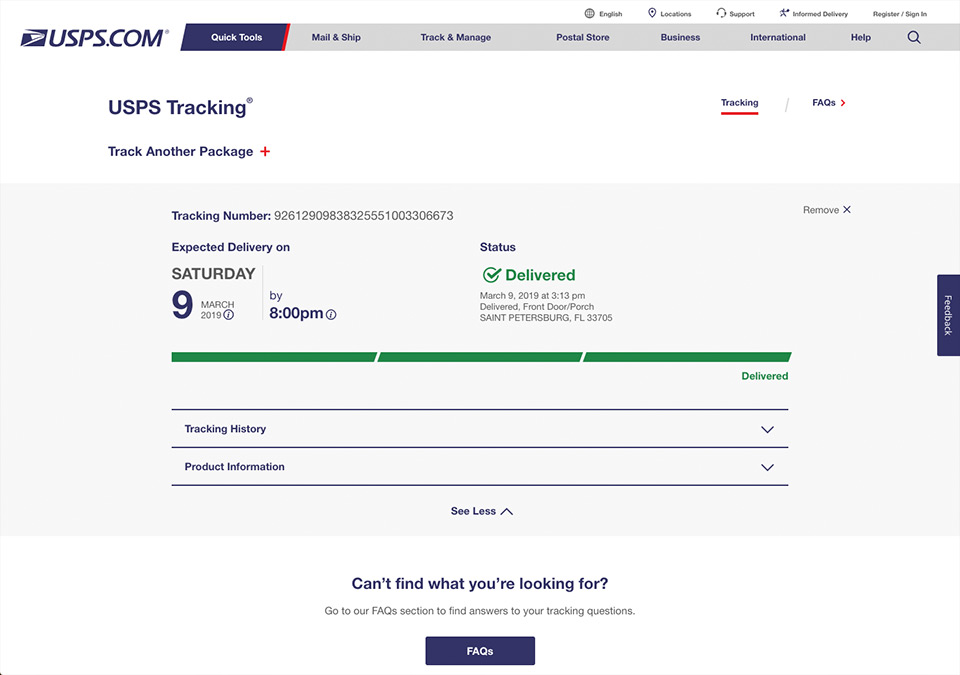The image displays a webpage from UPS.com. In the upper left corner, there is a UPS logo. To the right of the logo, there's a dark blue area labeled "Quick Tools." Further to the right, a gray bar contains several clickable options, which, despite being somewhat blurred, can be identified as "Mail & Ship," "Track & Manage," "Postal Store," "Business," "International," and "Help."

In the top right corner of the page, there are various settings and account options including "English," "Location," "Support," "Informed Delivery," "Register," and "Sign In." Below these options, the page focuses on package tracking, with headers for "USPS Tracking" and "Track Another Package."

The tracking details provided are for a package with the tracking number 9261-2909-8383-2555-1003-306673. The expected delivery was slated for Saturday, March 9, 2019, by 8 p.m. However, the package was delivered earlier, on March 9, 2019, at 3:13 p.m., to the front door/porch in St. Petersburg, Florida.